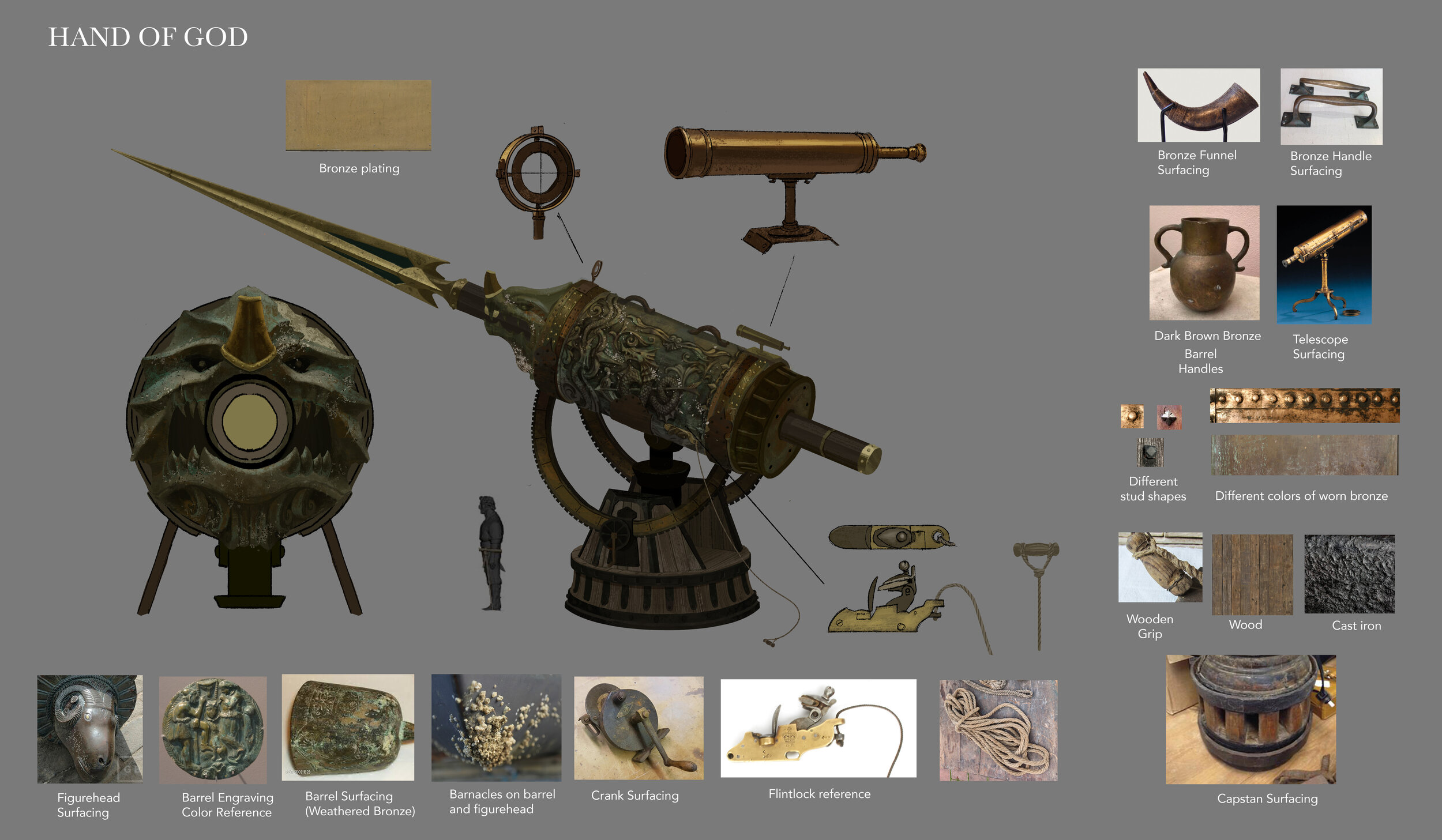The image showcases a detailed virtual exhibit titled "Hand of God" displayed against a light gray background. Dominating the center is an immense machine that resembles a catapult, sporting a large spear pointing towards the top left, reminiscent of a weapon, yet mounted on a base akin to a telescope stand. This towering machine looms over a human figure, hinting at its massive scale. Surrounding this central piece are numerous smaller images and photographs that display an array of objects and materials primarily related to bronze and metalwork. Notably, there are labeled images of a goat's head figurine titled "Figurehead Surfacing," as well as detailed photographs showing "barrel engraving," "barrel surfaces" in weathered bronze, and samples of different shades and textures of bronze and wooden grips. To the upper right and left of the main structure, there are images resembling a telescope and crosshair guides, respectively. The exhibit includes various unique artifacts like a funnel, a dark brown bronze barrel, and custom-made metal pieces, displaying the intricate craftsmanship involved. The overall arrangement suggests a focus on metal engraving and artistic creations, presenting a fascinating glimpse into the artistry of metalwork.